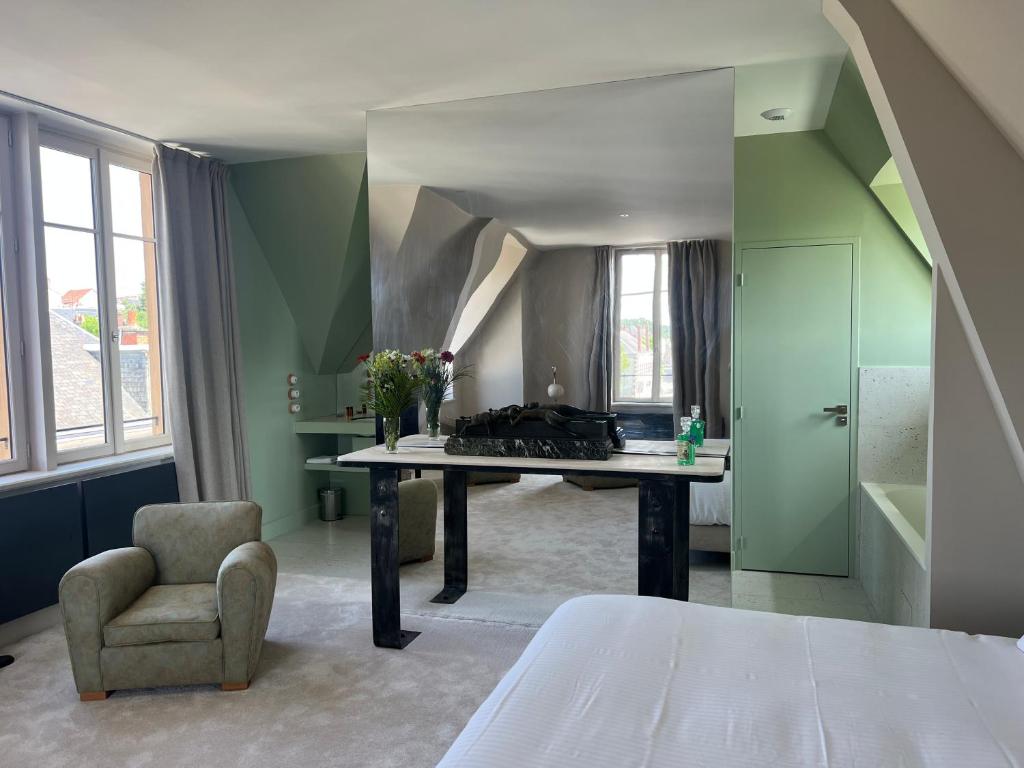The image depicts a well-lit, spacious room, possibly a hotel room or an unconventional bedroom, showcasing various distinctive features. The walls at the back are painted green, complemented by a white ceiling and white right-hand sidewall. The floor appears to be covered with off-white or gray carpet. Large windows adorn the left wall, with gray curtains partially drawn, offering a view of another building's roof. 

In the foreground, the right side reveals the corner of a bed with an unmade white sheet, and to the left, there's an armchair. A bathtub is positioned near the bed, close to a closed door on the right, which could be an entrance. The lower left corner of the room features a lounge chair and a small inlet with a possible trash can, countertop, or sink. 

Centrally placed in the room is a white table with black legs, surmounted by a substantial square mirror that reaches the ceiling. This mirror reflects the opposite side of the room, revealing gray walls and another window with matching gray curtains. This detailed image captures a unique blend of furnishings and spatial arrangement, creating an intriguing and somewhat eclectic room layout.